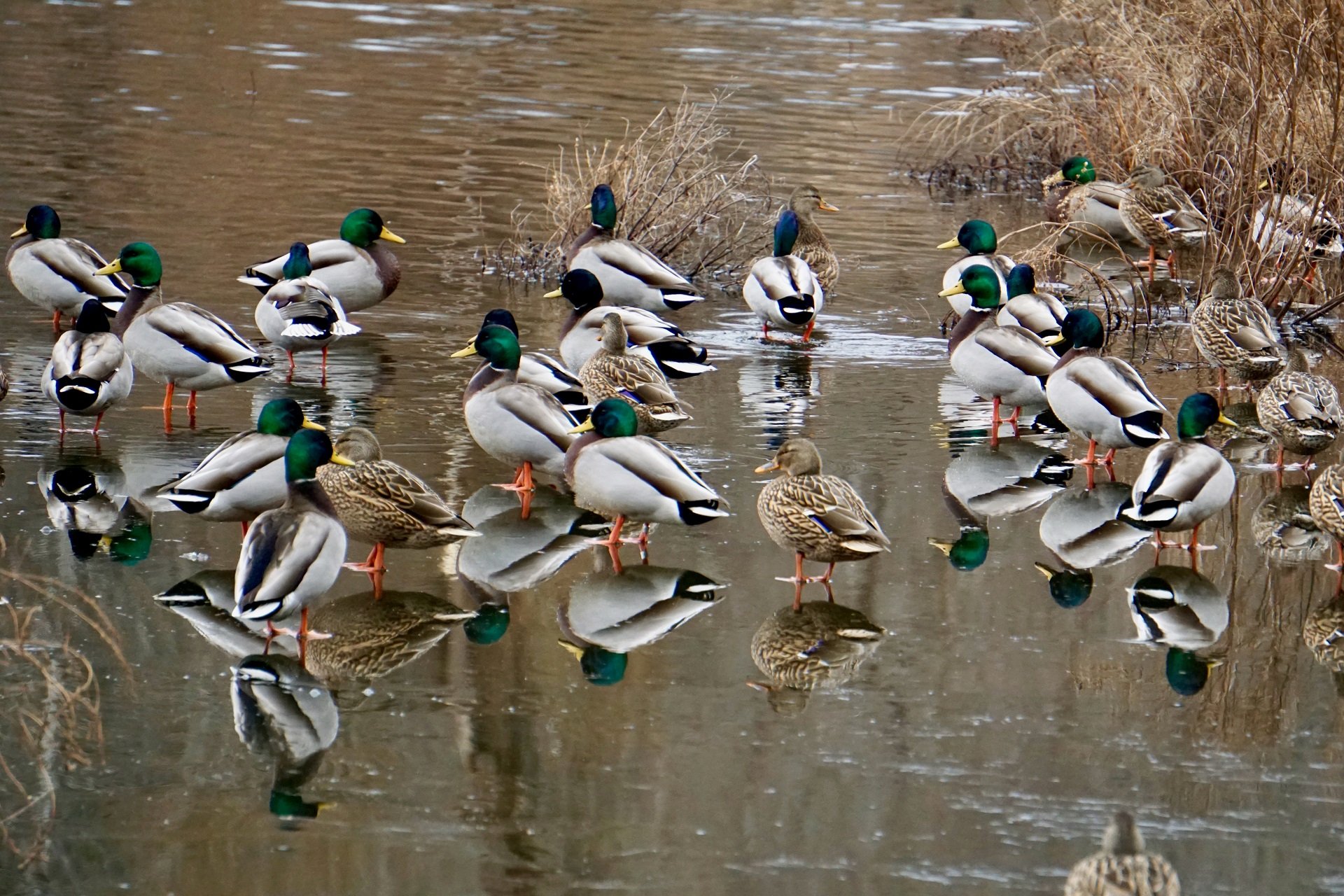This detailed photograph captures a large flock of mallard ducks wading in very shallow, murky gray water that could be a pond, lake, or marshy area. The majority of the ducks are males, distinguishable by their striking iridescent green heads and gray bodies with distinctive white rings around their necks, contrasted with their orange legs and feet. There are also several female ducks, marked by their more subdued brown plumage, scattered among the males. In total, there appear to be around 20 to 24 ducks, creating a lively scene with their various poses and reflections on the still water surface. Some males exhibit blue-toned heads, adding a touch of diversity to the flock. Surrounding the ducks and jutting up from the water are numerous dried, brown plants, indicative of a late fall or winter setting. The central positioning of the ducks against this natural backdrop emphasizes their vivid colors and tranquil demeanor as they wade and prepare to swim.